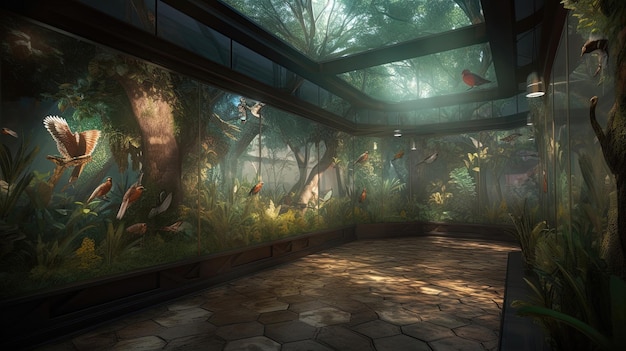A highly detailed mural resembling a panorama of a jungle environment, complete with vibrant depictions of birds and trees, wraps around the left side in an L-shape. The glass walls, extending from the ground to the ceiling, along with a glass roof, allow natural light to flood the space, adding to the realistic ambiance. The ceiling glass also showcases live green trees visible from outside, blending seamlessly with the mural. An orange-chested bird, possibly a robin, is perched near the skyline portion of the mural. Adjacent to this area, to the right, there appears to be a section resembling an aquarium, with the possibility of fish visible within. The scene is completed with a tiled floor and stone hexagonal panels spread throughout the main corridor, enhancing the exhibit's intricate design. This immersive setup, reminiscent of an indoor nature reserve or advanced concept art, captures the confluence of natural and artificial elements, making it a captivating visual experience.